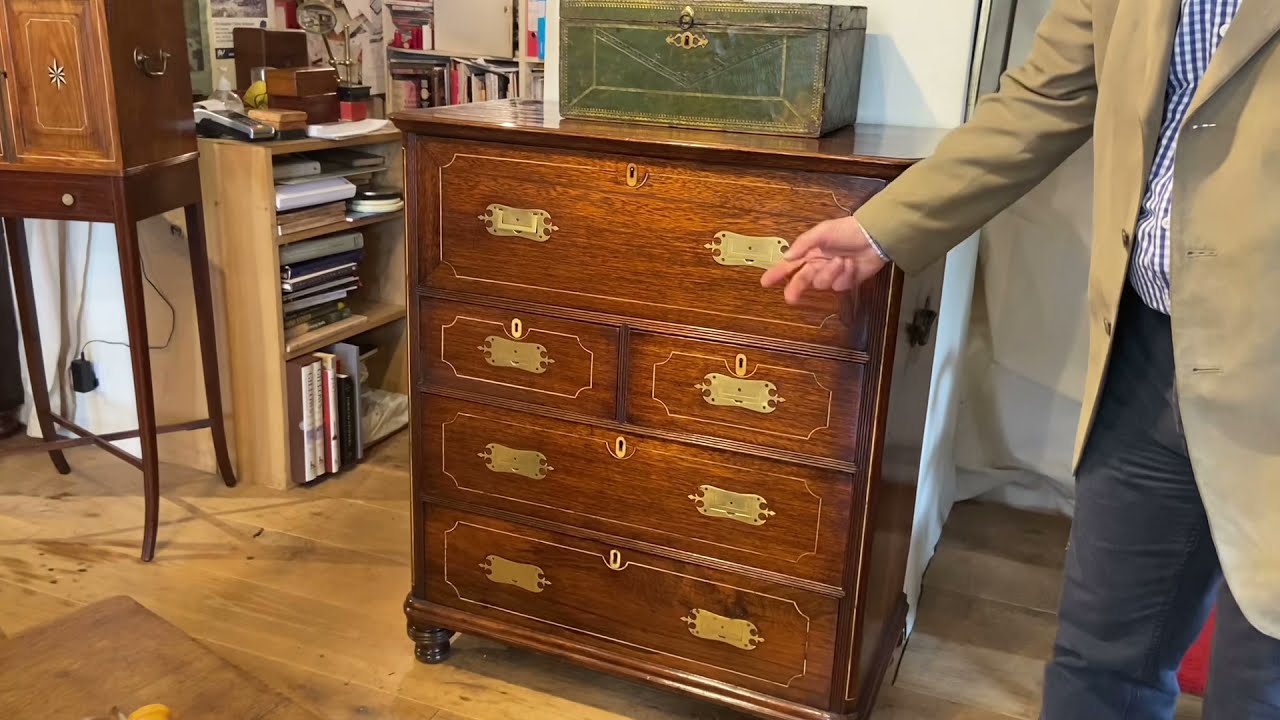The image showcases a richly hued brown dresser with a polished mahogany finish, positioned centrally on a hardwood floor. This dresser, characterized by its classic design and rounded knobby legs, features four rows of drawers with elegant gold handles and subtle keyholes. The top row is a single, spacious drawer, followed by two smaller drawers, an intermediate drawer, and another large drawer at the bottom.

Atop the dresser sits a vintage green lockbox, adding a touch of nostalgia to the setting. To the left of the dresser, there's a small shelf filled with books, and in the far left upper corner, a brown stand with another brown chest can be observed. Additionally, in between the dresser and the shelf, there's a glimpse into another room with more bookshelves laden with various items.

To the right of the dresser, partially in the frame, a man dressed in a tan sport coat over a blue and white plaid shirt with dark pants is prominently featured. His right hand points towards the dresser, drawing attention to its detailed craftsmanship and possibly the green lockbox on top. His gesture and attire suggest he may be explaining or highlighting something about the dresser, which appears to be in an office or a well-furnished room.